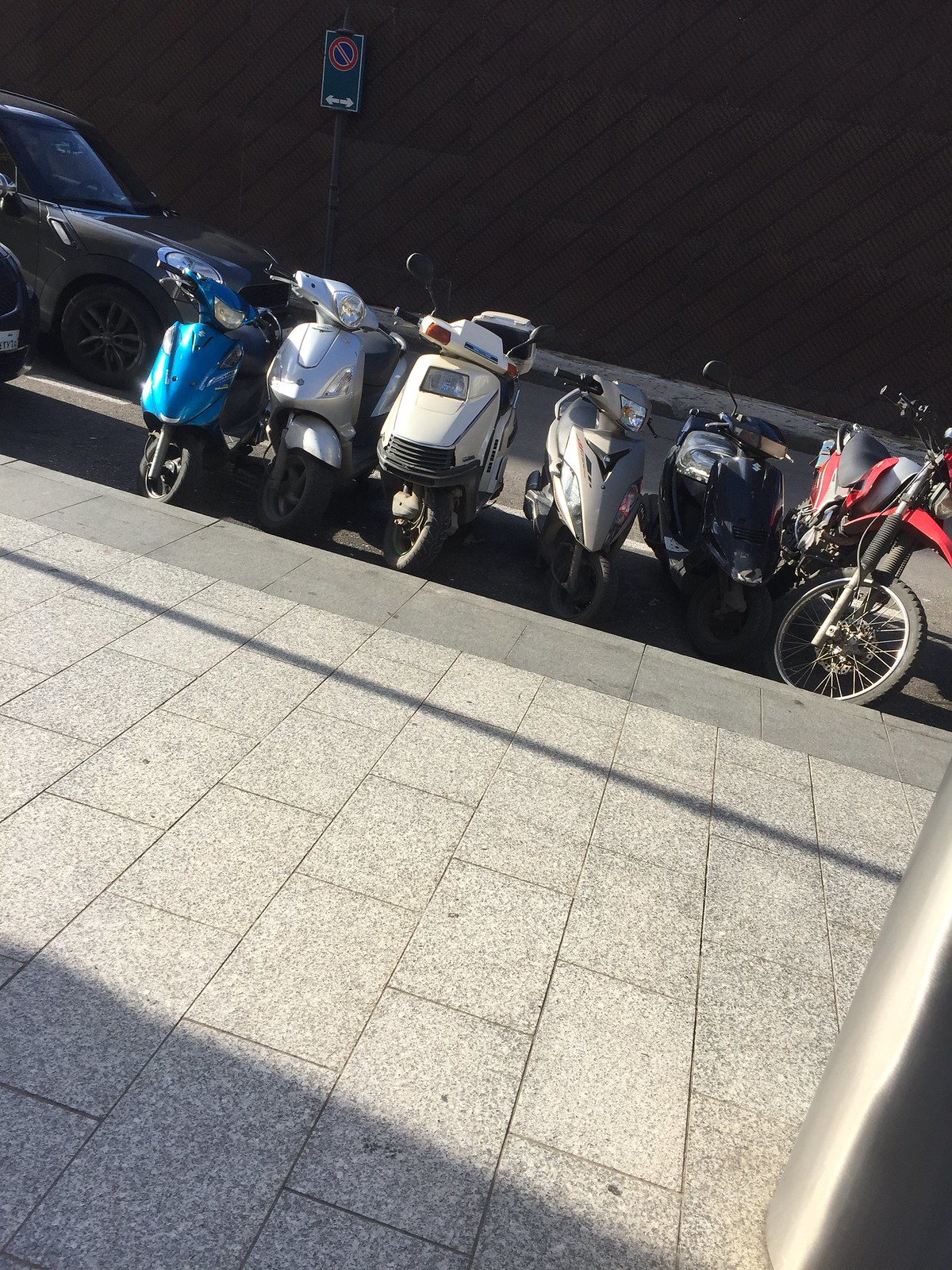The image depicts seven motorcycles lined up along a sidewalk with rectangular gray speckled tiles on a slightly downhill street. From left to right, the motorcycles include a blue one, another blue one further left but slightly hidden, a silver one, a white one with an older design, a gray one, a black one, and a distinctive red and black bike with a smaller front tire, resembling a moped. Behind the motorcycles is a black car that resembles a Mini Cooper, either parked or driving by. In the background, there's a big brown wall adorned with diagonal lines. There's also a visible sidewalk with a partial view of a metal pole nearby. Prominently displayed is a pole with a rectangular sign featuring a red circle with a cross through it and white bold arrows pointing in both directions, indicating no parking in the fire lane area. The scene is bright and sunny, capturing the bustling urban environment.